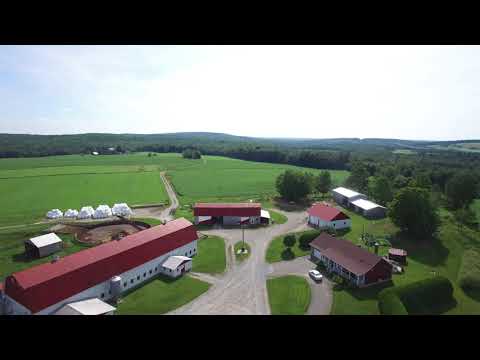This color photograph provides a detailed aerial view, likely captured by a drone, depicting a rural farm compound surrounded by expanses of lush green grass, fields, and tall trees. Central to the image is a long barn-like building adorned with a red metal roof and an adjacent silo, suggestive of agricultural activity. Directly across from this structure is a brown building featuring a U-shaped driveway, facilitating access to the main road. Adjacent to these is a smaller white building with a red roof, possibly a chicken house, accompanying another similar structure, each with tin roofs further in the background. A parked car is visible beside one of the buildings, highlighting the area’s scale. In the distance, the serene landscape transitions into rolling hills carpeted with greenery, under a pale sky that completes this panoramic farmland vista.